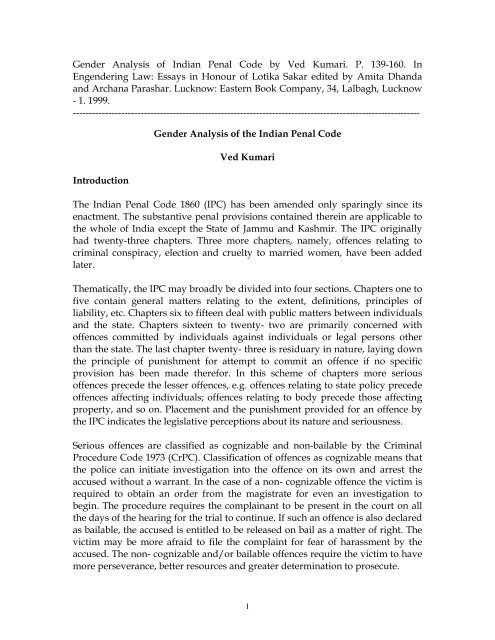The image shows a scanned, black-and-white front page of a study titled "General Analysis of the Indian Penal Code" by Ved Kumari, extracted from the publication "Engendering Law: Essays in Honor of Latika Sarkar," edited by Amita Danda and Arkana Prashar, and published by Eastern Book Company in Lucknow in 1999. The study covers pages 139 to 160 and introduces the Indian Penal Code (IPC) of 1860, highlighting its limited amendments and its applicability to all Indian states except Jammu and Kashmir. The IPC, originally comprising 23 chapters, has expanded to include additional chapters on offences like criminal conspiracy, election-related offences, and cruelty to married women. Thematic divisions are described across four sections: general provisions (Chapters 1-5), public matters (Chapters 6-15), individual offences (Chapters 16-22), and a residual chapter on punishment for unlisted offences (Chapter 23). Emphasis is given to the classification of serious offences as cognizable and non-bailable under the Criminal Procedure Code of 1973 (CRPC), detailing the differences in police authority and procedural requirements for cognizable and non-cognizable offences, as well as the challenges victims may face in prosecuting such crimes.